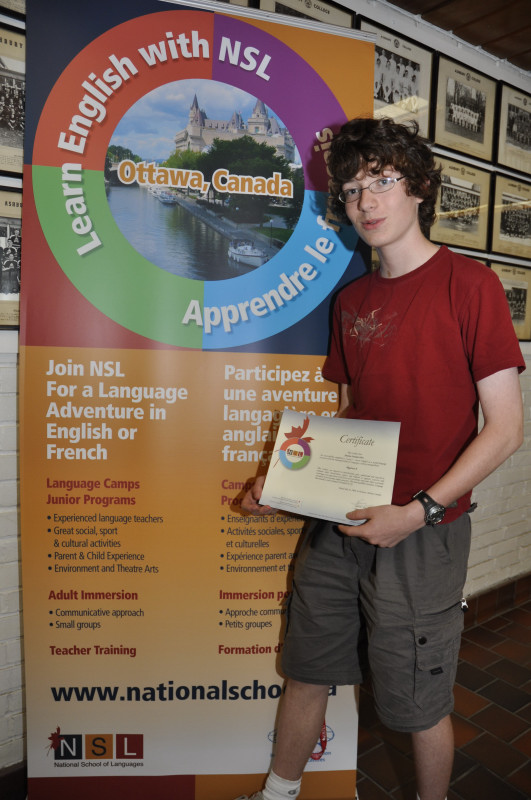In this detailed indoor photograph, a smiling teenager with short brown curly hair and glasses stands slightly to the right, directly facing the camera. He wears a red t-shirt, grey cargo shorts, and a wristwatch on his left wrist. Grinning proudly, he holds a certificate in both hands, positioned just above his waist. Behind him, a large rectangular poster occupies the left side of the image. The poster features a circular emblem at the top with an image of Ottawa, Canada, surrounded by colors including green, red, purple, and blue. Beneath the emblem, the text "Learn English with NSL. Ottawa, Canada" is prominently displayed, followed by details about language programs offered by NSL. The right column of text is partially obscured by the boy, but phrases such as "Join NSL for a language adventure in English or French," and further descriptions of various programs can be seen. At the bottom of the poster, "WWW.NationalSchool" and boxed letters "NS" and "L" are visible. The backdrop consists of a white brick wall adorned with numerous photo frames showcasing group photos of students. The setting, featuring a brown brick floor, is well-lit, suggesting it is midday inside a language facility.